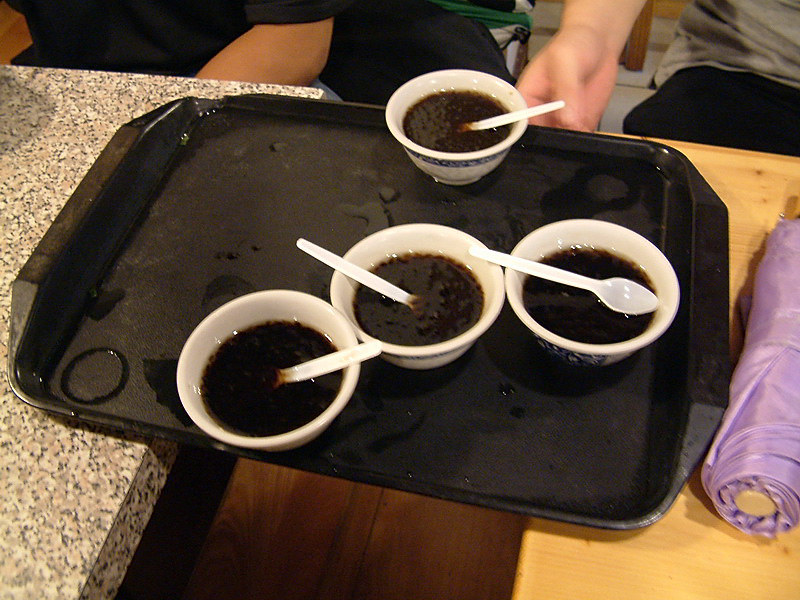In this digital photograph taken indoors, a black plastic tray with handles integrated into either side is positioned between two distinct tables. The tray stretches from the left, resting on a speckled granite-like surface with black, beige, and gray flecks, to the right, where it sits on a light-colored wooden table. The right side table features a folded lavender umbrella between the tray's end and the edge of the picture.

The tray holds four large white cups or small soup bowls, each containing a dark brown liquid reminiscent of French onion soup without the onions, or an au jus sauce. Each bowl has a white plastic spoon either placed inside or resting across the top. Notably, the spoons in the first three bowls are positioned differently: one facing right, another facing left, and the third also facing left but merely resting on the surface. The fourth bowl's spoon is submerged and facing right.

In the upper right corner, a person dressed in black pants and a green t-shirt reaches down toward the tray. Meanwhile, the upper left corner reveals part of a person wearing a black t-shirt and jeans, with their arm visible below the elbow. The scene appears to capture a moment in what could be a kitchen or restaurant, highlighted by the mix of marble and wooden surfaces and the casual placement of the individuals.